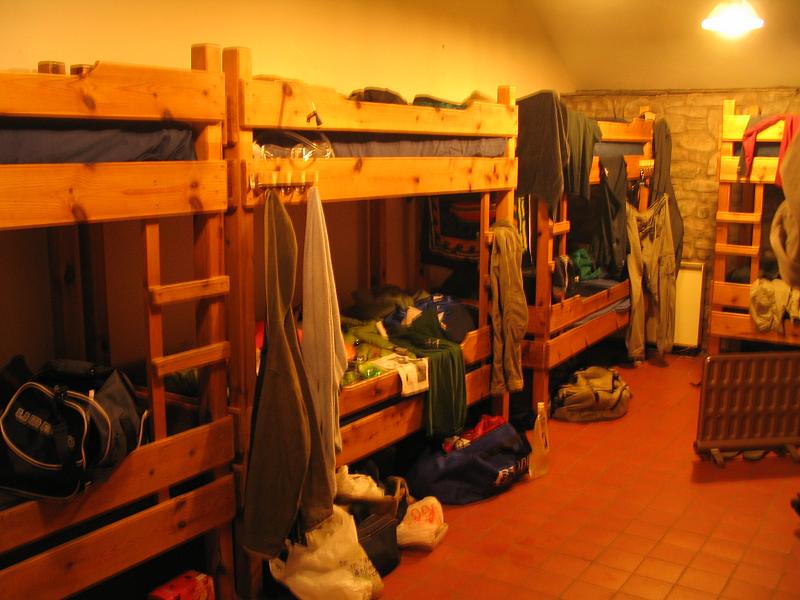This color photograph, likely taken inside a youth hostel, captures a dimly lit room with an overall orange-red hue. The room features a terracotta-colored tile floor and three visible bunk beds, handmade from light brown or walnut-stained wooden planks. These bunk beds are lined up along the left wall, beneath a cream-colored drywall that slopes toward the far right of the image. The far back wall showcases a patterned stone design.

Each bunk bed, appearing equipped with a built-in two-step ladder on the right, is adorned with gray overalls hanging from the top to the bottom. The beds are unmade, displaying messy sheets and an array of personal items such as duffel bags, backpacks, and sweatshirts scattered across the mattresses and the floor. Additional luggage items are present, adding to the cluttered appearance. The rightmost edge of the image reveals just a portion of another bunk bed, suggesting the continuation of similar structures along the back wall. Above this area, a yellow light softly illuminates the tan brick wall in the background.